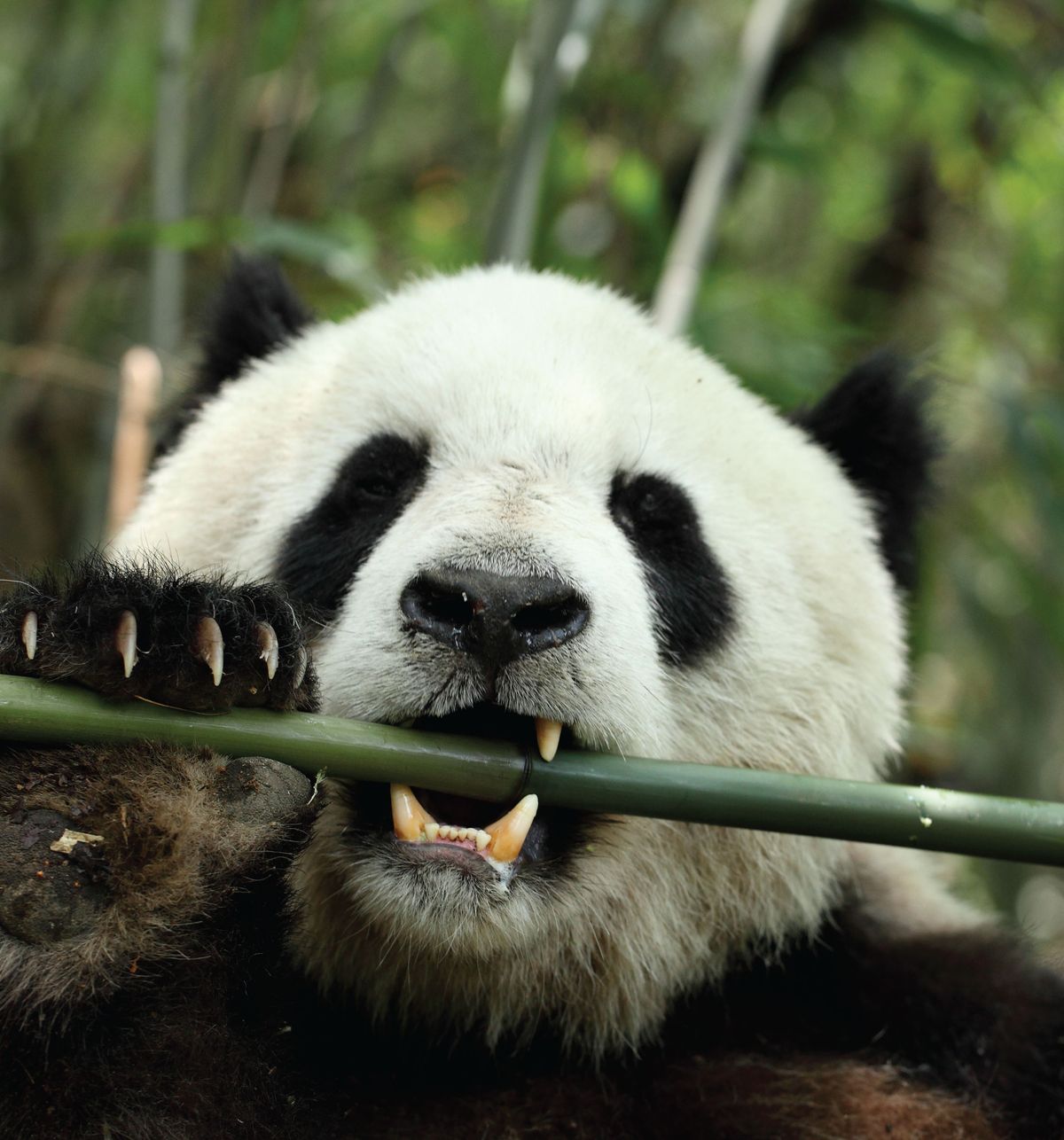This close-up photograph captures a panda in a natural setting, chewing on a dark green bamboo rod held horizontally in its mouth. The panda's face is predominantly white, with striking black patches around its eyes and a black snout. Its ears are black, matching the visible parts of its body and its black paws, which grip the bamboo. The panda's teeth, some of which are yellow, are visible as it bites into the bamboo rod. The claws on its paws are quite pronounced, featuring brown bases with tan tips. The background of the image is blurred, showcasing lush green foliage and bamboo stalks, enhancing the natural ambiance of the scene.